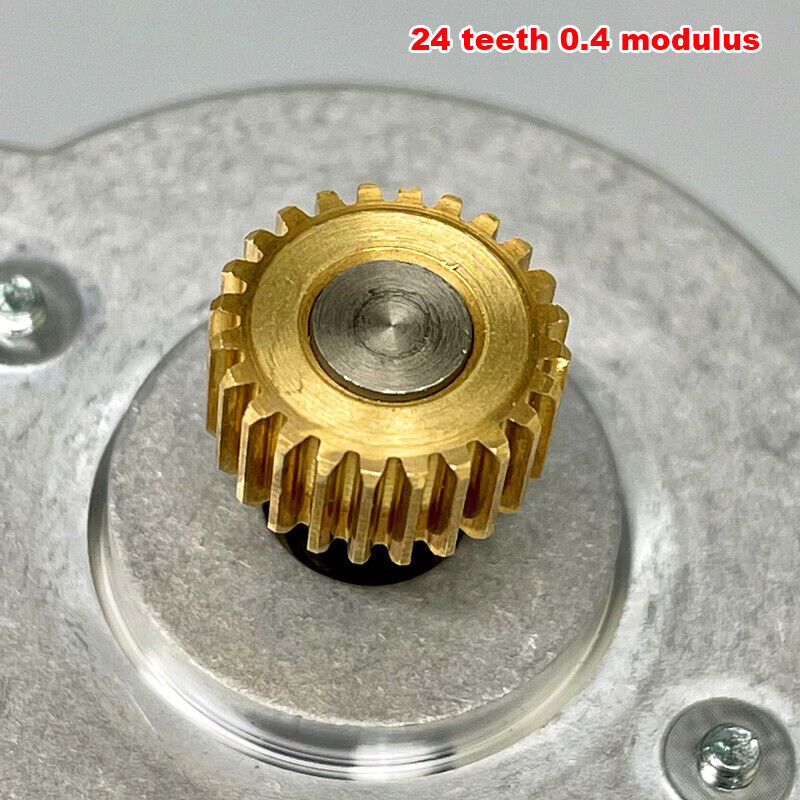This photograph, taken indoors, captures a detailed close-up of a mechanical gear assembly. The image is square, measuring approximately five to six inches on each side. The background is a steel gray color. Starting from the upper left and upper right corners, the image features a rounded faceplate that extends down by about an inch on the left and two inches on the right before curving upwards to meet in the center.

The faceplate itself, constructed from silver metallic material, slightly extends off-screen on its left, right, and bottom edges. Prominently visible on the upper left and lower right sections of the faceplate are two silver bolts with washers beneath them. At the center of the faceplate, there is a raised circular section with a black cylinder rising to meet a central gold gear. This gear measures roughly an inch and a half in both width and height. The gear’s center features a dark grayish-silver bolt.

In the upper right corner of the photograph, red text with a white outline reads, "24 teeth, 0.4 modulus." This text overlays the light gray background and provides technical details about the gear. The entire composition highlights the intricate details of the mechanical components, emphasizing the industrial design and precise engineering of the assembly.